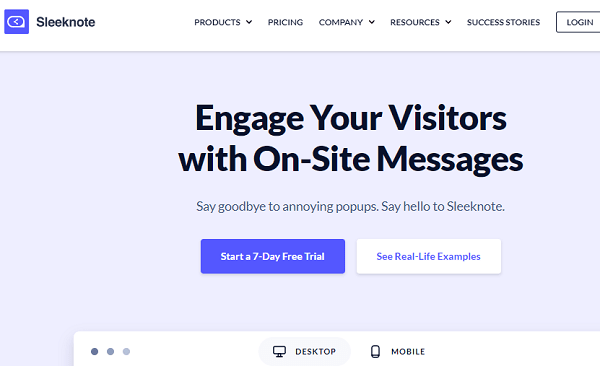The image features a promotional webpage for a product called "Sleek Note." 

In the top left corner, there's a sleek blue logo consisting of an arrow within a chat bubble. To the right of the logo, there's a horizontal menu with the following categories: "Products" with a downward arrow indicating a submenu, "Pricing," "Company" with a downward arrow, "Resources" with a downward arrow, and "Success Stories." Further to the right, there's a "Log In" button separated by a vertical line.

The main headline of the page reads, "Engage your visitors with onsite messages. Say goodbye to annoying pop-ups. Say hello to Sleek Note." Beneath this headline, there's a prominent blue button with white text that reads, "Start a 7-day free trial." 

Adjacent to this button is a white box with blue text labeled "Mobile," accompanied by an image of a phone. To the right of the phone image, there's another white box with blue text labeled "Desktop," situated next to an image of a computer monitor. The entire image has a clean, white background.

Overall, the image presents a clear, user-friendly interface designed to promote Sleek Note's services, highlighting their mobile and desktop compatibility.